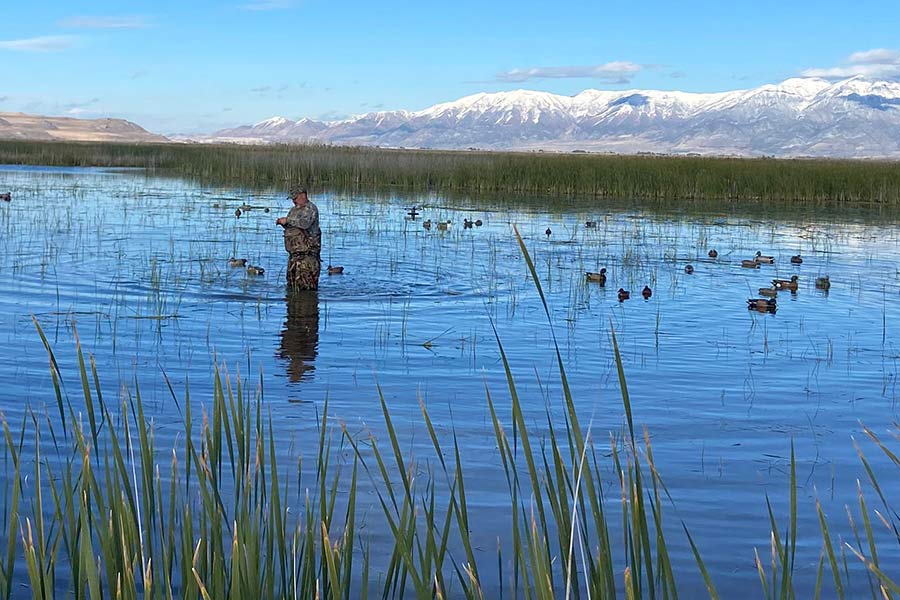A serene daytime scene captures a fisherman standing knee-deep in the calm, blue waters of a wetlands area, dressed in camouflage attire, complete with a hat. The foreground is dominated by tall reed grass, framing the tranquil setting. Ducks float peacefully in the water around the man, who appears to be fishing. In the distance, majestic snow-capped mountains rise up to touch the few clouds in the clear, blue sky. The overall atmosphere suggests a peaceful, possibly windy day in early spring or summer.